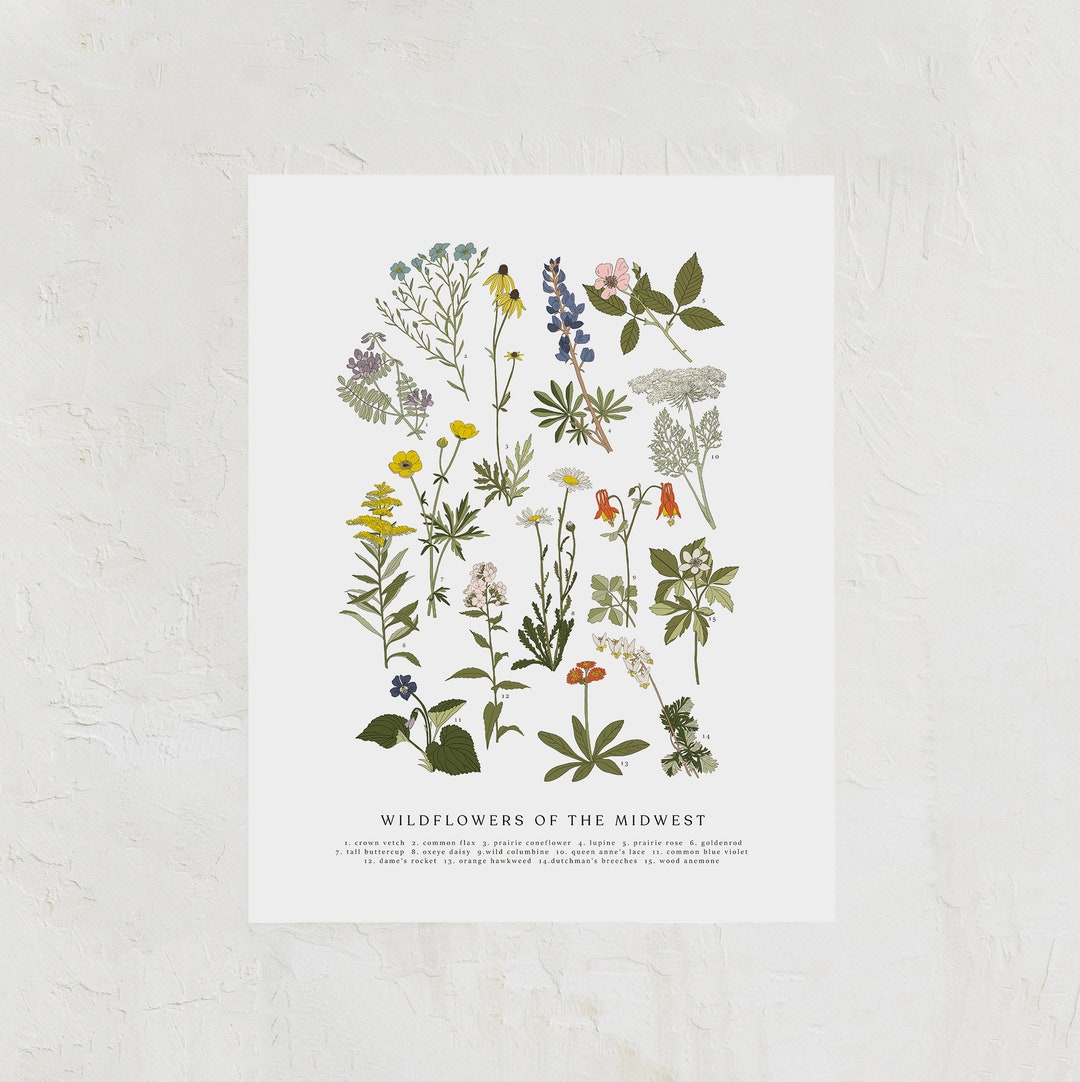The image is of a centered photograph of a poster featuring hand-drawn wildflowers, against a white, textured stucco wall. The detailed artwork highlights a variety of Midwest wildflowers with an array of vibrant colors including light blue, bright yellow, lilac, pink, and orange. Among the flowers depicted are blue petals resembling bluebells or lilies, conical yellow daisies, pink flowers with large petals, and white Gerbera daisies. Other flowers include deep dark blue blooms with large leaves, dainty white flowers, and passionate orange ones. At the bottom of the poster, the title "Wildflowers of the Midwest" is written in a serif font. Below this title, small numbered labels correspond to the names of each flower type, although the text is too small to be read clearly.